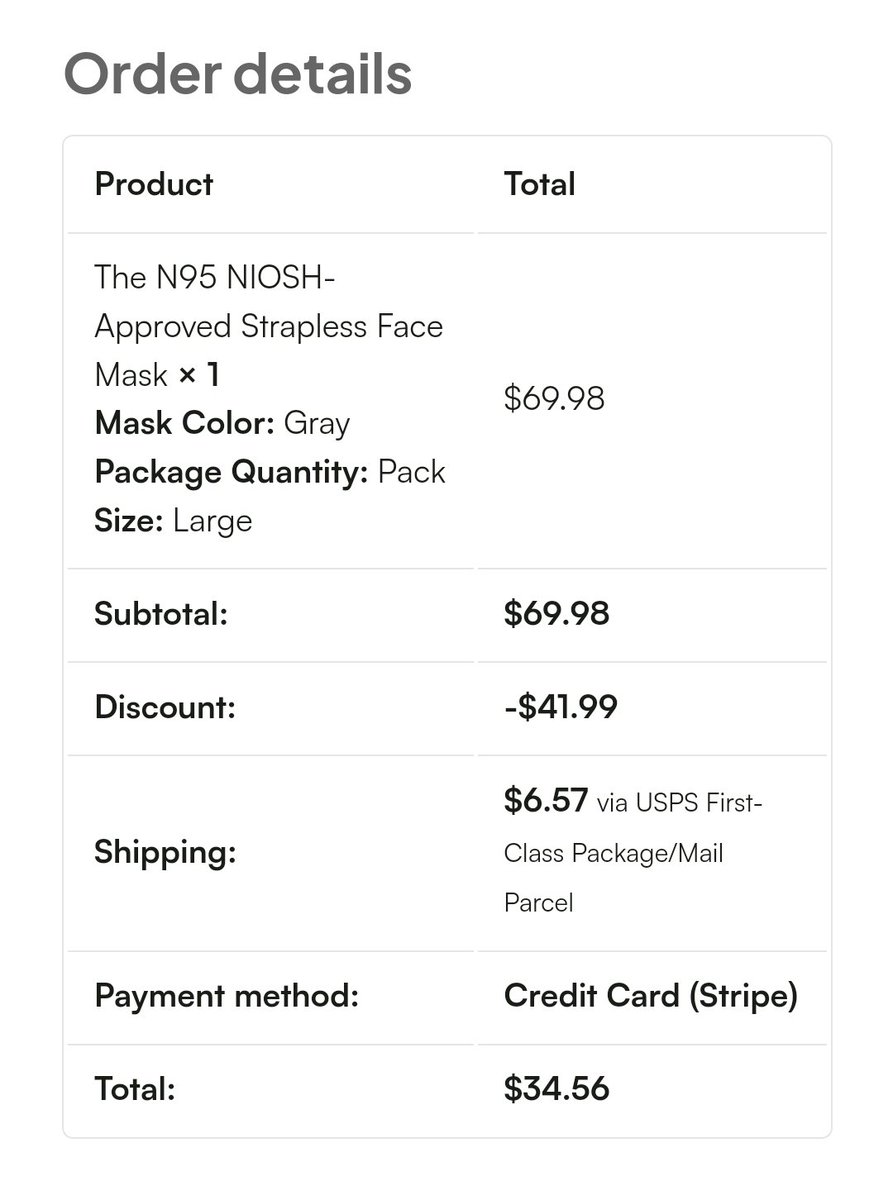Detailed Caption:

"A customer has purchased a high-quality, hospital-grade N95 NIOSH-approved strapless face mask. The mask, designed to filter out small particulates, is a resilient gray color and comes in a large size. Initially, the subtotal for purchasing a single mask was $69.98. However, after applying a significant discount, the total dropped to $34.56. This includes an additional shipping cost of $6.57, sent via USPS First Class Package. The transaction was completed using a credit card. The mask, known for its rigorous standards, offers superior protection compared to regular fabric masks commonly used during the COVID-19 pandemic."